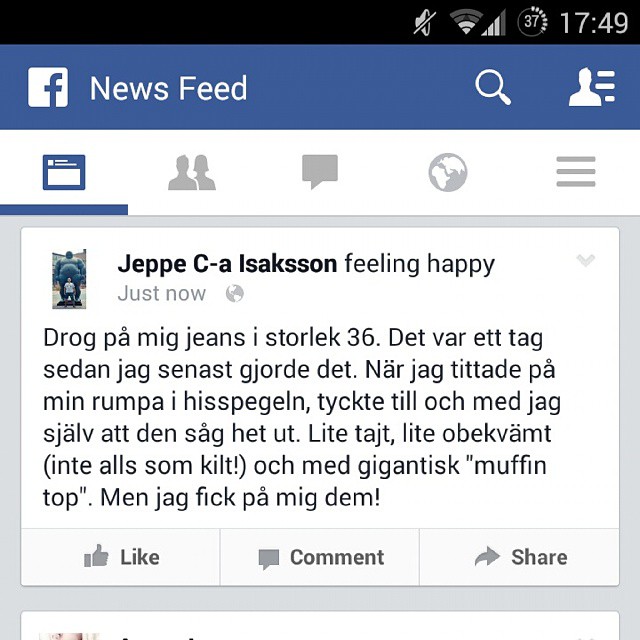📱 Jeff C.A. Isaacson is feeling happy

Just now, Jeff posted a new status on Facebook, featuring a unique image. The post shows Jeff standing in front of a large statue, possibly a Buddha, which can be slightly seen in the background. The interface displays multiple familiar icons like a thumbs up for like, a comment bubble, and a share arrow. 

The status message itself is written in a foreign language using Roman or Latin letters. Jeff shares that he managed to wear a pair of pants, expressing a mix of surprise and amusement. Despite feeling a bit uncomfortable and commenting on his “muffin top,” he is happy he could put them on. 

Additional details captured include a timestamp of 17:49, with Jeff’s device showing a battery life of 37% and two bars of WiFi. The sound for the device was off at the time of the post. 

👍  💬  🔁